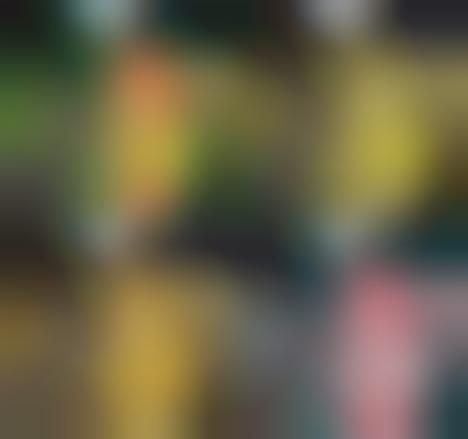The image depicts a young girl with red hair and white skin wearing a yellow shirt and brown overalls, standing next to a gray baby goat with tan features. Both are set in an animated landscape featuring green hillsides, flowers, pine trees, and a cloudy sky. This scene is presented in four squares, where the initial image in the top left corner remains unaltered, while the subsequent three are modified with varying filters and differing saturations, changing the tints and colors of the original. Notably, the girl's hair color shifts from orange to brown, tan, and reddish hues across the images. Similarly, the girl's outfit and the baby's goat features undergo subtle color adjustments. Each image has different captions at the bottom right corner: "Normal," "Protein Poppy," "Junior Topic," and "Triton Topic," respectively.